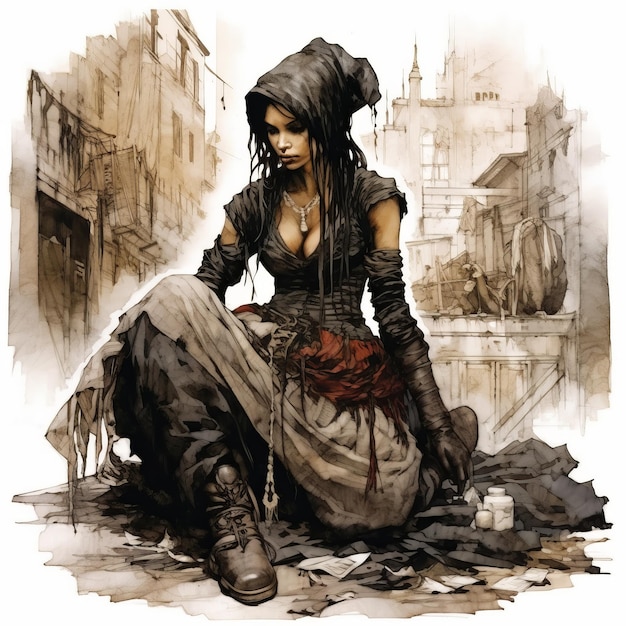In the center of the image, a woman with long dark hair sits amidst what appears to be handmade art, possibly based on an actual photograph. She is dressed in a Gothic Victorian style outfit featuring a black corset and matching black gloves that extend nearly to her shoulders. A gray or silver necklace adorns her exposed cleavage. Her attire includes black boots and a dress which, due to its length and folds, gives the impression of black pants as she sits with her legs crossed. She dons a dark black hood and is looking downward with a melancholic expression. Surrounding her is a pile of black fabric, under which newspapers are partially visible, along with a couple of pill bottles to her right. The background shows the outlines of gray, water-colored buildings with sepia and beige tones, sketchily rendered to blend with the white outline encircling her, emphasizing the delicate balance between her and the backdrop.